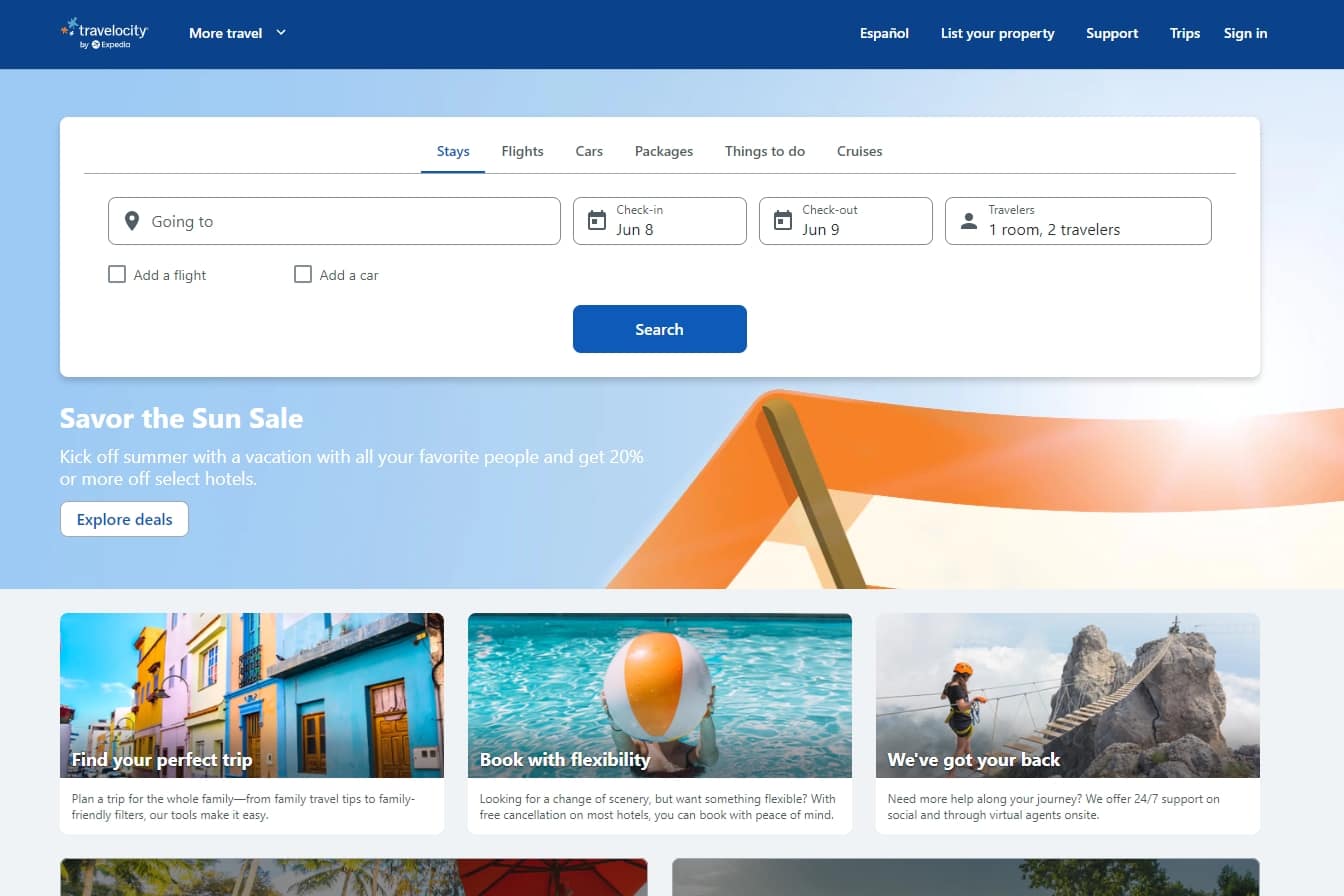The screenshot captures the homepage of the Travelocity website. The header is set against a blue background, featuring the Travelocity logo alongside the white text "Travelocity by Expedia." To the right of the logo, bold white text reads "More travel" accompanied by a pull-down menu. Further to the right, options in white text include "Español," "List your property," "Support," "Trips," and "Sign in."

Below the header, a light blue banner displays the text "Savor the sun sail," encouraging users to "Kick off summer with a vacation with all your favorite people and get 20% or more off select hotels." Above this promotional message, a white search bar prompts users to enter their destination with the placeholder "Going to." The search bar also includes fields for "Check-in" and "Check-out" dates, which are preset to June 8th and June 9th, respectively, and an option for "Travelers," set to one room and two travelers. 

Beneath the search bar is a blue action button labeled "Search." Below this button is a section displaying an image with overlaying text that reads "Find your perfect trip," featuring icons of a city street, a beach ball representing "Book with flexibility," and a person in a pool.